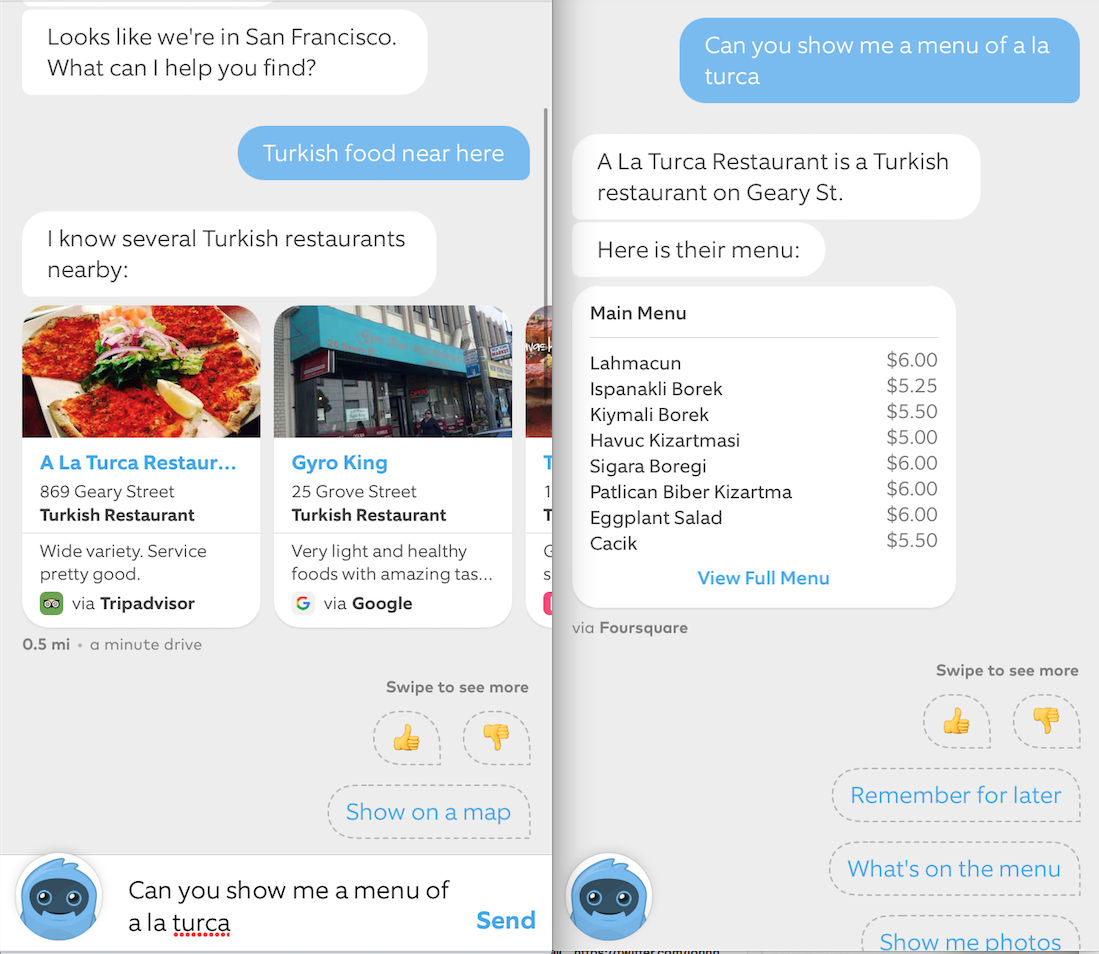This image shows a detailed screenshot of a chat interaction within the Foursquare application. The conversation begins with a message from the chat box stating, "Looks like we're in San Francisco. What can I help you find?" The user responds with, "Turkish food near here." The chat box replies, "I know several restaurants nearby," and suggests two options: Alaturka Restaurant and Garo King. The user then asks, "Can you show me a menu of Alaturka?" The chat box provides information about Alaturka Restaurant, noting it is located on Geary Street, and displays part of its menu.

The menu is titled "Main Menu" and features the following items:
1. Lahmacun - $6
2. Ispanaklı Börek - $5.25
3. Kıymalı Börek - $5.50
4. Havuç Kızartması - $5
5. Sigara Böreği - $6
6. Patlıcan Biber Kızartma - $6
7. Eggplant Salad - $6
8. Cacık - $5.50

At the bottom of the menu, there is an option to "View Full Menu." This screenshot provides a clear view of a user seeking out Turkish cuisine and getting detailed menu information from an AI chat within the Foursquare app.